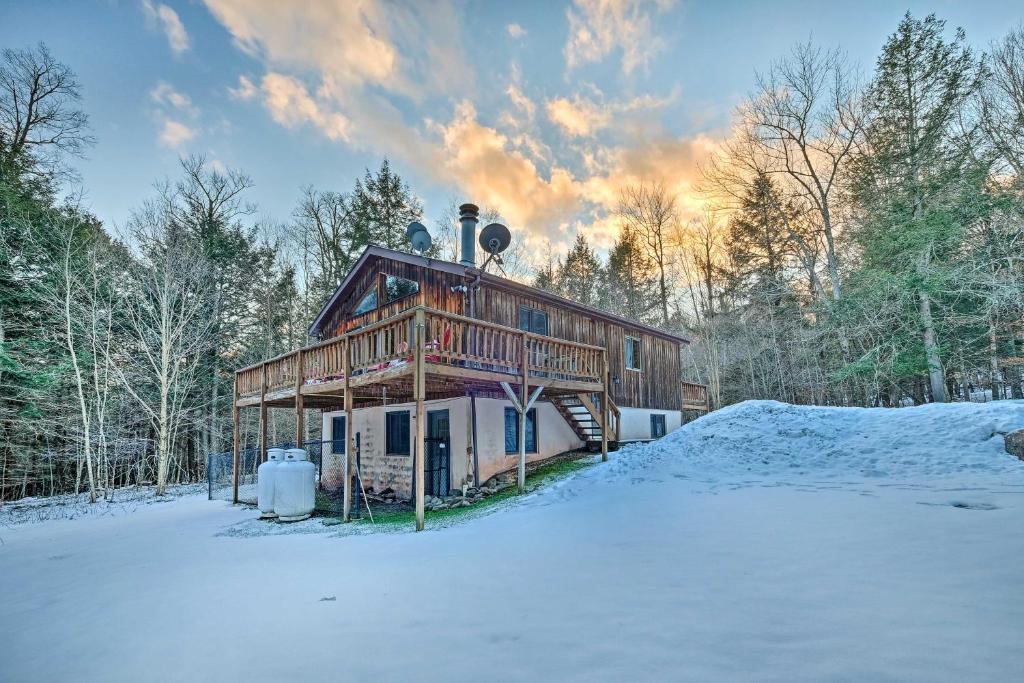The image depicts a rustic dark brown cabin nestled in a forested area, bathed in the soft hues of sunset. The sky exhibits a gradient from blue to a pinky orange as the sun dips behind the evergreen and bare deciduous trees, including aspens and quakes. The cabin, with vertical wood siding and a beige foundation, features a wide wraparound deck on the second level that can be accessed by steps on the right-hand side. Two tall, white propane tanks stand prominently in the front yard beside a large mound of snow, which, along with scattered patches, blankets the ground. The roof hosts two—or perhaps three—satellite dishes and a metal chimney centrally located between them. A water catchment system is visible at the front of this two-story home, embodying a blend of rustic charm and practicality amidst its serene wintry setting.